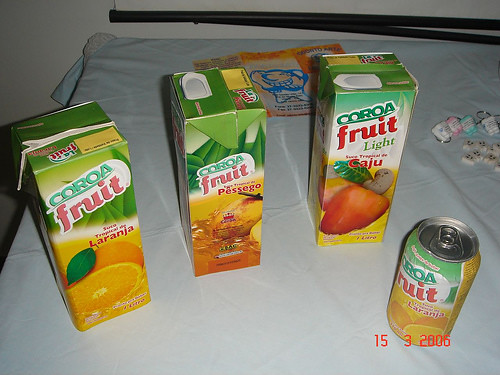This image showcases an assortment of fruit juice containers displayed on a table covered with a slightly wrinkled white tablecloth. Positioned prominently in the lower right-hand corner is a 12-ounce aluminum beverage can with green and yellow graphics, labeled "Carroja Fruit Laranja." Centrally, the image features three branded aseptic boxes. The leftmost box is labeled "Carroja Fruit Laranja" and displays an image of an orange, indicating the flavor. The middle box reads "Carroja Fruit Pasego," likely peach, with a corresponding fruit image, while the rightmost box is labeled "Carroja Fruit Light Kaju," featuring a fruit image that might represent cashew apple. All containers share the same design elements, emphasizing the brand "Carroja Fruit." In the background, a few small, unidentifiable objects are scattered, including a brochure. The image was captured on March 15, 2005, noted as "1532005."